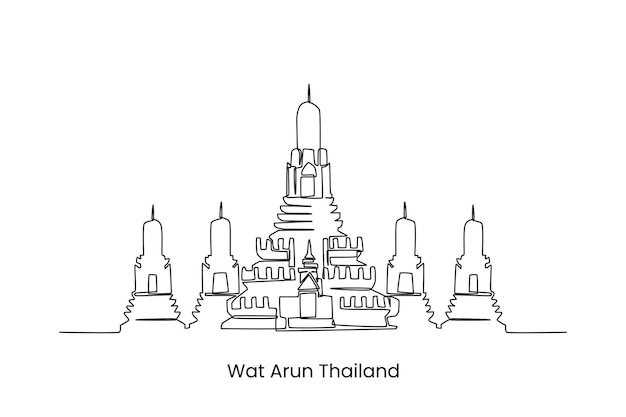The image is a detailed, monochromatic pencil drawing on a white background, depicting Wat Arun, a significant temple in Thailand. The temple is centrally placed, with the main structure being the tallest and most ornate, emphasizing its importance. The main building is flanked symmetrically by two smaller structures on each side. Each temple features distinct shapes and scintillated layers reminiscent of castle walls, with doorways and zigzag patterns adding to the intricate design. The tops of the buildings are rounded, tapering off to points resembling straight lightning rods. This artistic drawing, likely created by a computer or AI due to its precise line work, uses a single unbroken line to outline the temples, adding a modern touch to the traditional subject. The title "Wat Arun, Thailand" is inscribed at the bottom, making it recognizable as an iconic representation of this famous Thai landmark.